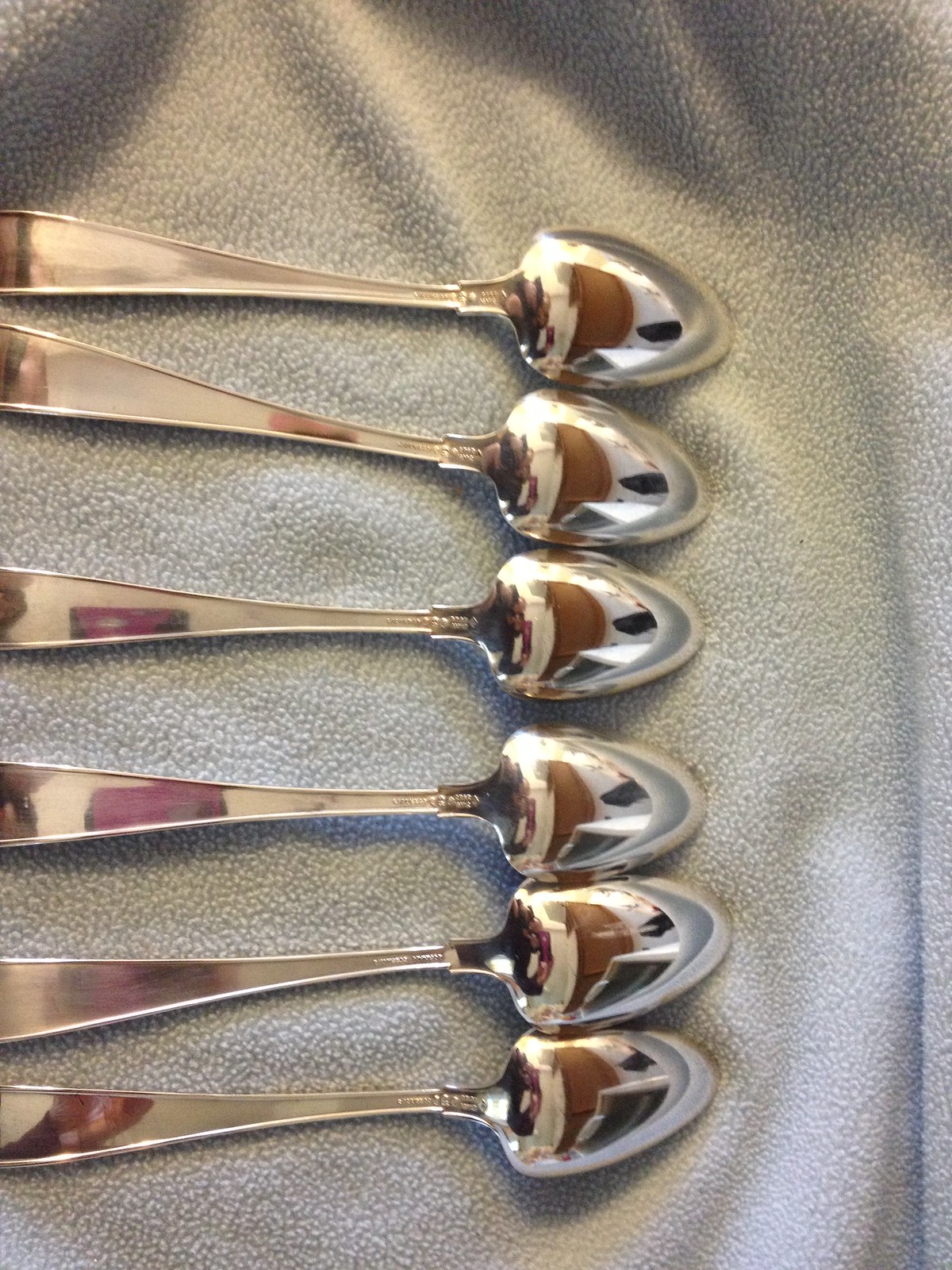This photograph showcases six highly polished silver spoons meticulously arranged upside down on a gray microfiber cloth, possibly an anti-tarnish fabric often used to wrap silverware. The handles of the spoons are all aligned to the left, while the bowls extend to the right of the image, their shiny surfaces reflecting intricate details. The back of the spoon bowls reveals reflections of a brown cabinet, a burgundy object, and even the person taking the photograph, holding up the camera. A hint of writing appears on the upside-down handles, suggesting they might be sterling silver, given their bright, vivid reflections and polished appearance. Shadowy areas at the top of the cloth add depth to the composition.